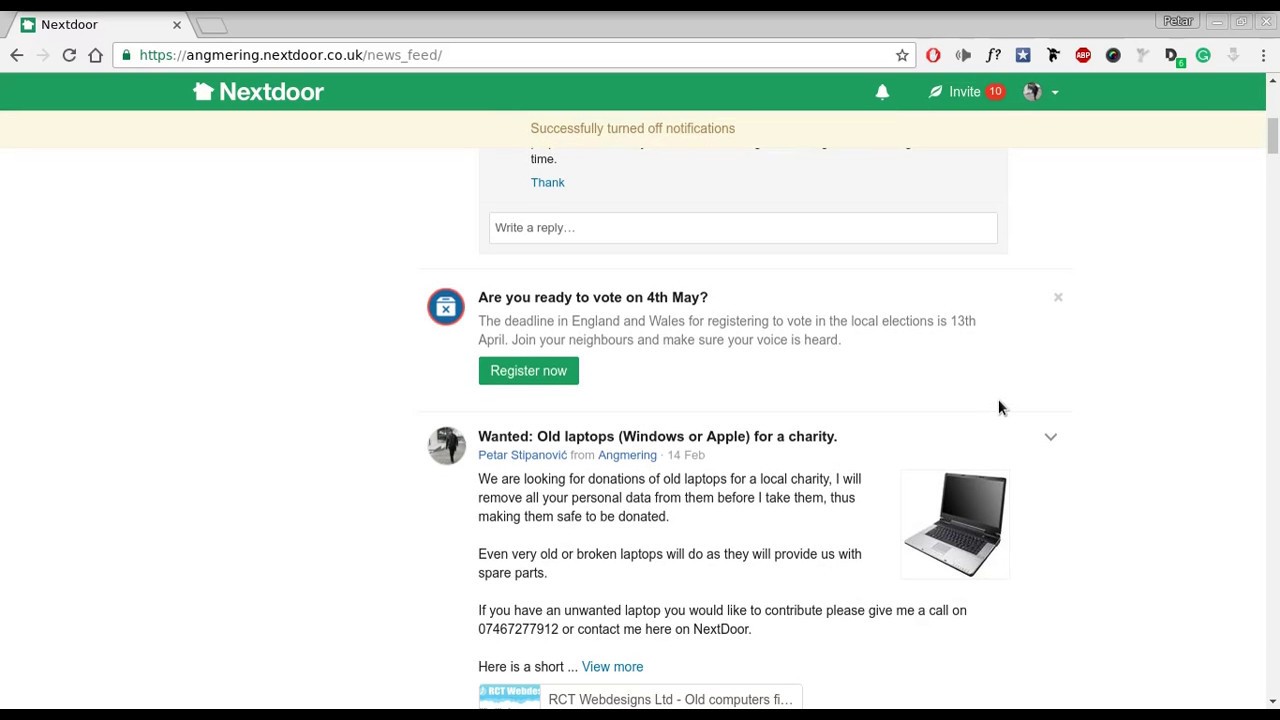The image depicts a web browser interface with detailed elements. At the top is a solid black line spanning the entire width. Below it lies a gray border, also extending across the page. An active tab, shaded light gray, prominently displays the text "next door" in black.

Across the top, the header reads "PETAR." The background features a web browser showing a URL in green: "https://", followed by "angmering.nextdoor.co.uk/news_feed" in black, with the underscore and other elements in gray. A green border appears beneath the URL, with "White House" and "next door" in white text next to a white bell and a white leaf. The word "invite" is also in white, and a red circle with a white "10" suggests notifications.

A potential profile picture, enclosed in a circle, is visible, though its contents are unclear as it appears in black. The background transitions to light yellow, featuring the text "We turned off notifications" in light brown. Below, there's a partial gray box with visible text, indicating the time and words "thank" and "tell," followed by "write a reply" in black.

Further down, the content asks, "Are you ready to vote on May 4th?" and informs readers about the registration deadline for local elections in England and Wales, set for 13th April. A call to action suggests joining neighbors to ensure their voices are heard. Below this is a green box with a "register" prompt in white. The image ends with a notice seeking old laptops for charity, stating the intent to remove personal data for safe donations, and welcomes both very old or broken laptops for parts.